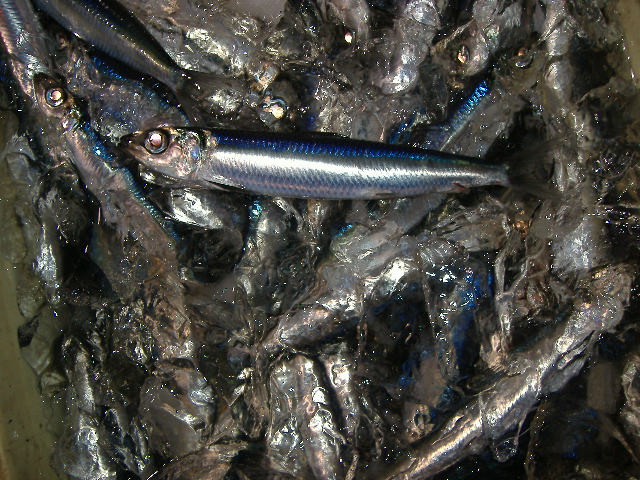The photo depicts a grim scene of several small fish, likely minnows or sardines, that have washed up on the shore and are now lying lifeless within a slimy, gooey mass. The fish are intertwined, one on top of another, making it difficult to distinguish individual features amidst the tangle. Their bodies exhibit a striking coloration with blue spines and silver bellies, and their large eyes and protruding fins are clearly visible. The slimy substance beneath them may be a product of decomposition, adding to the dismal appearance of the scene. Although one fish appears more vibrant than the others, perhaps indicating it died more recently, they all share the same unfortunate fate. The setting lacks any additional context or text, allowing the viewer to focus solely on the sorrowful clustering of these vibrant yet lifeless aquatic creatures.